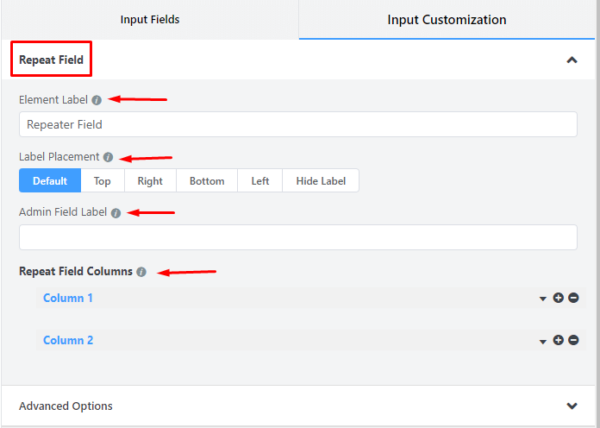This annotated screenshot appears to be of a user interface for an application focused on customizing input fields. The image seems to be a cropped section of a larger interface. At the top, there are two tabs labeled "Input Fields" and "Input Customization," with the "Input Customization" tab underlined in blue, indicating it is the currently active tab.

At the very top of the panel, the text "Request Field" is encircled in red. Directly below this, a red arrow points to an element labeled "Element Label." Adjacent to this label, there's a blank text box meant for user input, currently displaying the placeholder text "Repeater Field."

Further down, another red arrow points to "Label Placement," which offers six options: Default, Top, Right, Bottom, Left, and Hide Label. The "Default" option is currently selected.

Below this, a red arrow annotation points to "Admin Field Label," accompanied by another blank text box for text input, which at this moment is empty.

The next annotation points to "Repeat Field Columns," which contains two columns, "Column 1" and "Column 2," both highlighted in blue. To the far right of these columns, there is a drop-down menu followed by a plus (+) symbol and a minus (-) symbol for presumably adding and removing columns.

Lastly, at the very bottom of the image, there is a section labeled "Advanced Options" with a drop-down arrow, indicating that additional settings can be expanded if needed.

This detailed caption deciphers the various elements and annotations present in the interface.